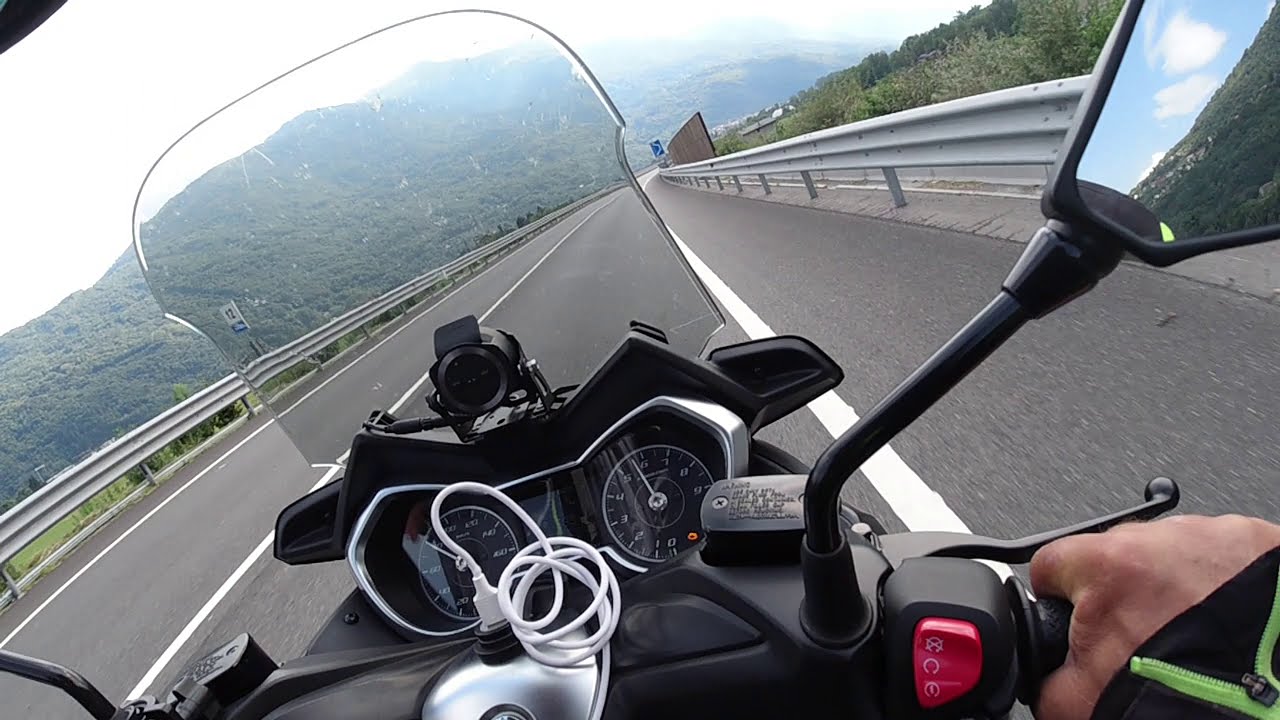This image, taken from the first-person perspective of a motorcycle rider during the daytime, vividly showcases a scenic mountainous highway. The rider, identified by a Caucasian hand gripping the throttle, is wearing a long-sleeve black jacket with a green zipper. Directly in front of them, a red button for the start and stop of the engine is visible to the left of the throttle. The right has a side view mirror reflecting a striking backdrop: a clear blue sky with scattered white clouds, and verdant green hills receding into the distance.

Centrally positioned on the motorcycle is a windshield, behind which lies an array of instrumentation including the speedometer, odometer, and a dash-mounted video camera. A white cord is connected, implying a charging device, possibly for a phone, plugged into the center console near the gas tank area. The two-lane highway ahead is marked by a single white stripe down the center and edges, flanked by metal guardrails on both sides. The surroundings exude natural beauty with expansive green mountains covered in grass and trees, under a resplendent sky. The road appears deserted, ensuring a tranquil ride for the solitary motorcyclist. The scene is rich with natural hues including blacks, greens, browns, grays, and silvers, punctuated by the vivid blue sky and the bright red switch on the motorcycle, perfectly capturing the essence of an adventurous journey through nature.